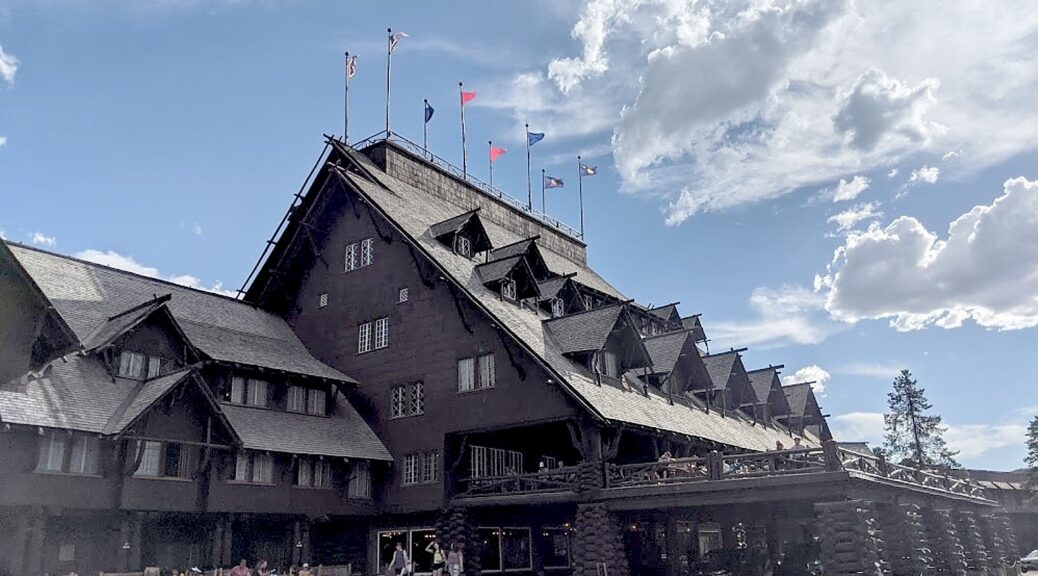The photograph showcases a large, elaborate building that strongly resembles a ski resort or mountain lodge. The building is distinguished by its dark gray or possibly faded black exterior and its geometric design, with multiple triangle-shaped roofs extending from a central, massive triangular structure. The structure appears to have between three to five floors, with many of the upper floors integrated into the sloping roof. 

The roof is adorned with six or eight flags, whose details are indiscernible, and illuminated by two lights. The ground is cropped out, making it unclear if there is snow present. However, a slight touch of snow seems to be dusting parts of the roof. The façade features large, open glass windows, particularly on the lower levels, allowing a view of the interior and the guests walking around.

A significant architectural highlight is the large porch or balcony on the second floor, supported by logs meticulously stacked like Lincoln logs, suggesting an elaborate, rustic style. This space is equipped with tables and chairs, likely serving as an outdoor dining area, possibly connected to a restaurant. Adjacent to this main building is a smaller structure with a similar design. The scene is set against a clear blue sky, dotted with fluffy white clouds, indicating a bright, cold day.